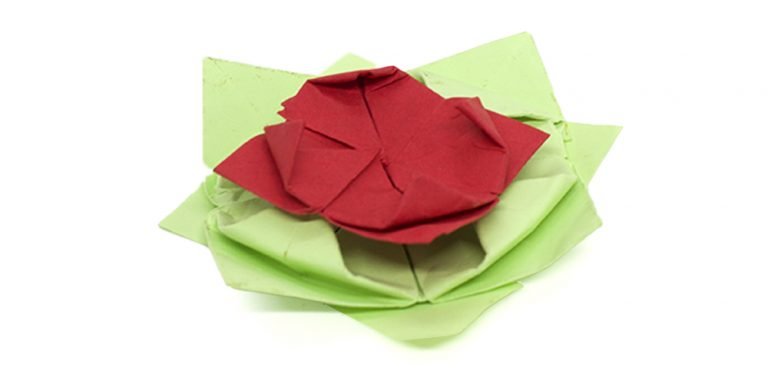This free-floating photograph on a stark white background captures an intricate origami-like arrangement of folded fabric napkins, creating a visually appealing piece of art. At the base, three light green napkins are meticulously layered in alternating directions, forming a leaf-like pattern. These napkins are folded in triangular and square shapes, with their edges neatly turned inward. Atop this leafy foundation, two red napkins are artistically placed, enhancing the design. The bottom red napkin is oriented in a diamond shape and lies flat, while the top red napkin's edges are slightly folded, resembling the petals of a flower. The overall composition, centered on the white background, uses layers and folds to create a harmonious blend of colors and shapes, with subtle shadowing adding depth and dimension.